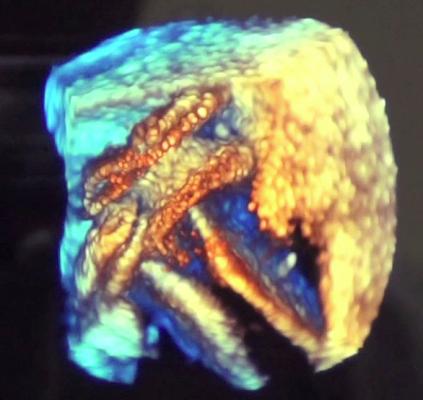This image features a highly detailed and vibrantly colored depiction of a mineral or stone set against a completely black background. The photograph itself is nearly square, just under three inches high and a bit over three inches wide, with slight raised areas on the left suggesting the background might be a folded black cloth.

The central subject is a roughly cubic block of stone, showcasing a variety of vivid colors. On the left side, at the top, the stone displays an electric light blueish-green tone that transitions into deep blues as it descends. The middle section features striking diagonal bands of gold intermixed with deep blues, creating a dynamic interplay of colors.

As you move to the right side of the stone, the colors shift dramatically to a bright, vibrant yellow, accentuated by dark streaks running through it, almost as if the light is illuminating this side from within. The topmost part of the stone features a color reminiscent of the Caribbean sea—a light bluish-green hue.

The bottom of the stone appears chipped and uneven, with some dark indentations that blur into the background, adding to the rugged texture and natural aesthetic. This intricately detailed image allows a view into the stone's interior, revealing different materials and textures that contribute to its overall striking appearance.